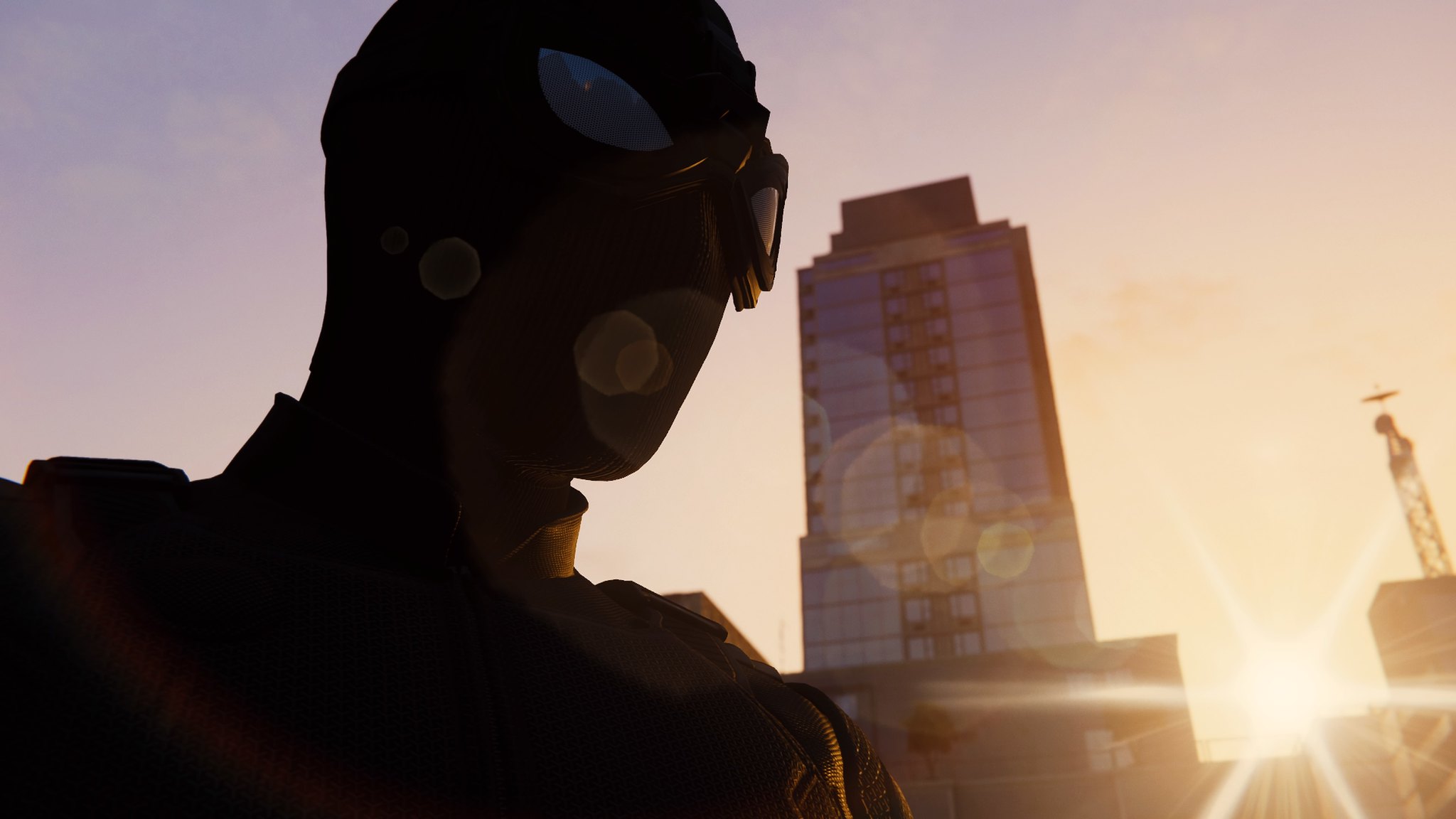The image appears to be a scene from a video game featuring Spider-Man. On the left-hand side, a character dressed in black is partially visible. His face is obscured by a mask, complemented by goggles with design elements reminiscent of Spider-Man’s eyes, featuring black rims and white centers. This character is gazing towards the right of the frame. He also wears a dark shirt, though the details are obscured.

In the bottom right corner, the sun casts a warm glow across the entire scene, creating a lens flare effect. Behind Spider-Man is a building adorned with blue windows, and to the far right, there is a radio tower. The sky transitions from a clear blue in the top left to a more yellowish hue near the bottom right, blending beautifully with the sunlight.